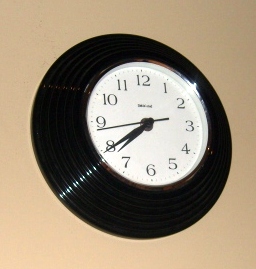This image features a detailed color photograph of a black-rimmed wall clock mounted on a beige wall. The clock's white face displays black numbers from 1 through 12 and has black hands, including a second hand positioned just below the 9, indicating the time is approximately 7:39. The clock’s rim is shiny and has a multi-layered, wide design with ridges, similar to the concentric grooves of a vinyl record, giving it depth and an interesting outward-angled appearance. There is a slight glare of light reflecting off the clock's glossy surface, creating a white line. The brand name on the clock face is not legible due to its small size.